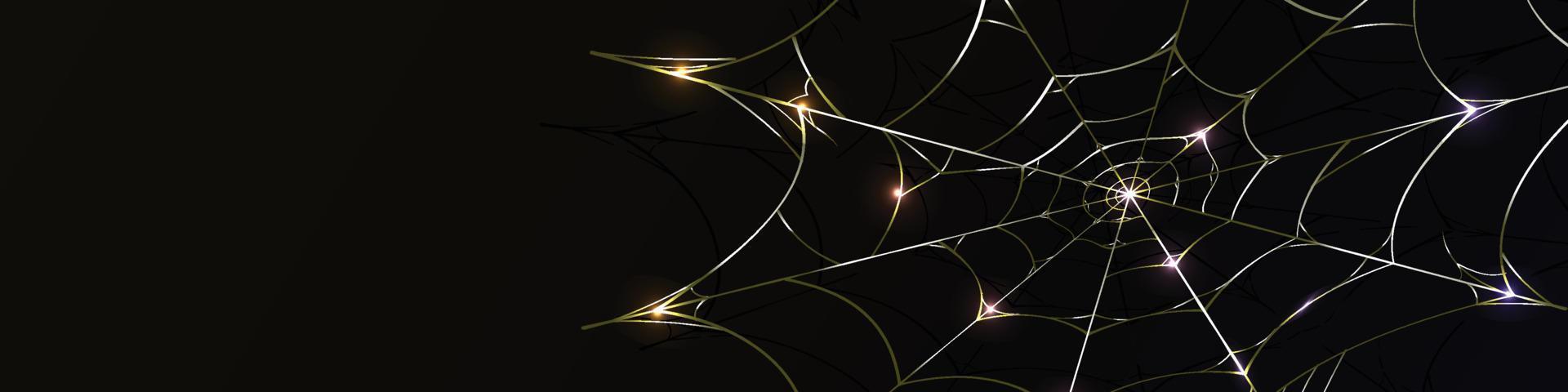This striking, rectangular image features a highly detailed, AI-generated spiderweb set against a pure black background. Occupying just over half of the right side of the landscape-oriented frame, the web is beautifully intricate, with layers that radiate outwards from a lit center. This center gives the web an appearance of light rays emanating from it. The web itself is depicted in varied hues, with sections appearing whitish-yellow, gold, and silvery, almost metallic and sparkly in nature. Despite its near-perfect geometry, the spiderweb has incomplete strands, making it look more like an artistic interpretation than a realistic spider's creation. The left side of the image remains completely blank, emphasizing the web's luminous and ethereal quality against the dark void.